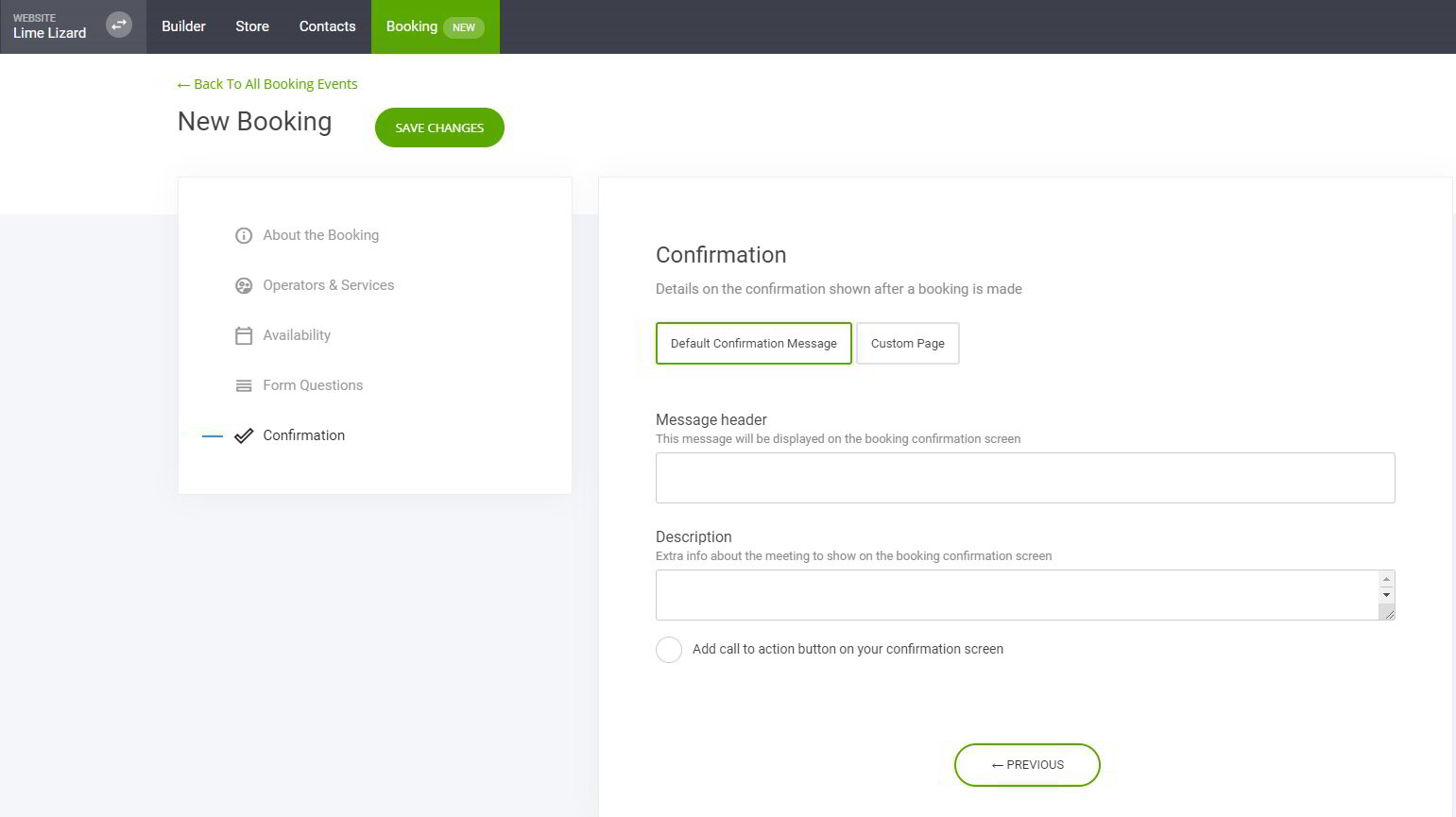This screenshot appears to capture the user interface of a booking management system. Dominated by a gray background with white typography, it features a central green section containing booking details. On the left, "Lime Lizard" is prominently displayed, accompanied by icons including arrows and circles, suggesting navigation options and builder/store contacts.

At the top of this section, a green banner reads "Back to all booking events" with a left-pointing arrow, followed by a gray text option "New Booking". Below these is a green button labeled "SAVE CHANGES" in all caps, written in white font.

The left sidebar lists several categories, each accompanied by a relevant icon:
- About the Booking
- Operators and Services
- Availability
- Form Questions and Confirmation

The main content area on the right starts with the word "CONFIRMATION", followed by an explanation: "Details on the confirmation shown after a booking is made" and "Default Confirmation Message," which is outlined in green. Below this section, a gray text option reads "Custom Page."

Next, there are fields for "Message Header," indicating space for a personalized message to be displayed during booking confirmation, and below it, a "Description" field for additional meeting information. Both sections include white text boxes for input.

Another feature in this area is a checkable circle labeled "Add Call to Action Button on your confirmation screen."

Towards the bottom center of the screen is a navigational button outlined in green, labeled "PREVIOUS" with a left-pointing arrow.

This comprehensive layout allows for detailed customization and management of booking events, including confirmation messages and additional meeting information.